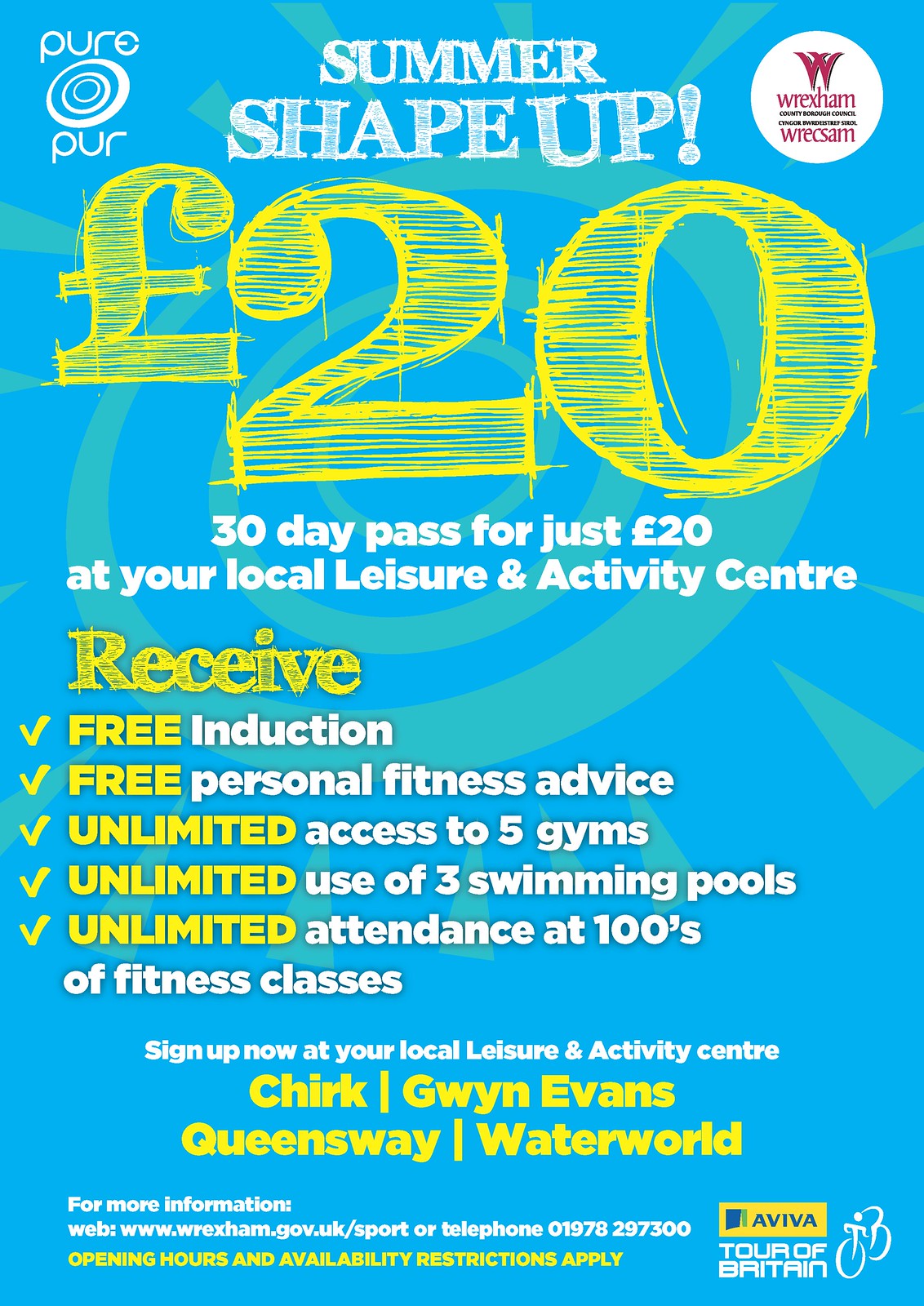This image is an advertisement for a local leisure and activity center's Summer Shape Up program. The background features a tealish blue color. At the very top, in white, capital letters with an exclamation point, it says "SUMMER SHAPE UP!", using a sketch-like, colored-in font style. Below that, in much larger, bold yellow lettering, it states "£20". Beneath the price, in white, normal font, it reads "30 day pass for just £20 at your local leisure and activity center." Following this, in yellow letters similar to the price text, the word "Receive" is highlighted, and a list of offerings is provided:

- Free induction
- Free personal fitness advice
- Unlimited access to five gyms
- Unlimited use of three swimming pools
- Unlimited attendance at hundreds of fitness classes

Each of these benefits is marked with a check mark, with the words "free" and "unlimited" emphasized in bold yellow text. Towards the bottom of the image, further contact information and signup details are provided, along with an image of a bicycle and the mention of "Aviva Tour of Britain" at the very bottom left. Additionally, it mentions "Shirk Gwen Evans, Queensway Water World" as part of the sign-up details.